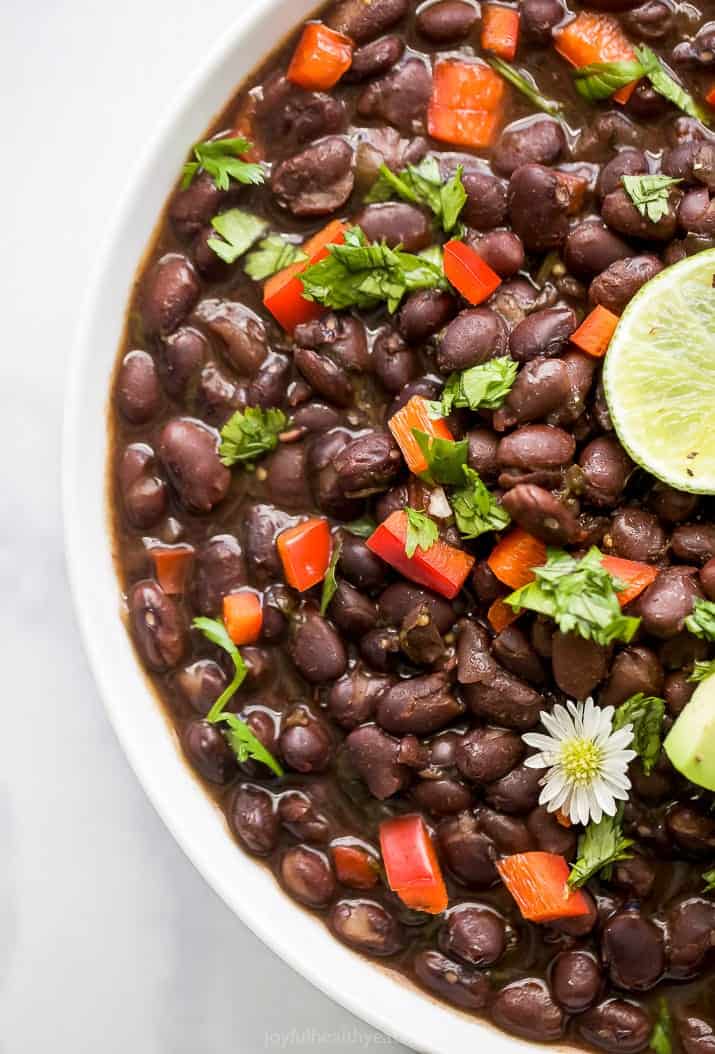This color photograph, oriented in portrait mode, offers a detailed view of a large white bowl containing a visually appealing dish of soupy black beans. The bowl, displayed only in its left half due to cropping, reveals a medley of ingredients that evoke a sense of a summer, possibly Mexican, recipe. The black beans are whole and submerged in a savory, broth-like liquid, resembling the consistency of chili or stew. Among the black beans, there are finely chopped red peppers, and bits of fresh cilantro scattered throughout, adding vibrant color and texture to the dish. Additionally, the bowl is garnished with a small white and yellow daisy and a half-visible lime slice placed towards the middle and upper right side. The bowl sits on a light gray background, highlighting its earthy, hearty presentation and aiming at a realistic, food photography style.